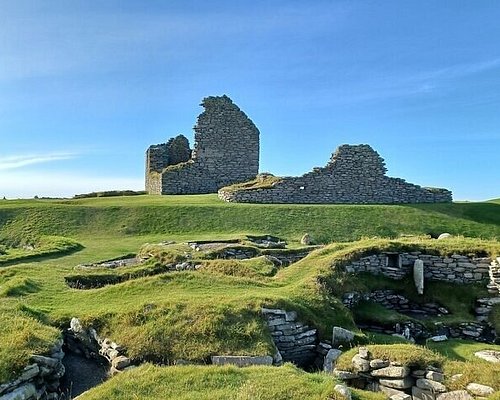The photograph captures a scenic ruin, likely situated in England or Scotland, against a backdrop of a clear blue sky with a few wispy white clouds. Dominating the background is a large, partially collapsed stone structure, possibly the remnants of a multi-story castle, built from light gray and white stones. This imposing ruin sits atop a flat-topped, grass-covered hill, lending an air of historic grandeur to the scene.

In the foreground, the gently rolling hills host additional stone buildings nestled into the landscape, with sections of their stone walls still standing. These buildings appear to use the natural contours of the hills, featuring grass roofs that blend seamlessly with the surrounding terrain. Scattered among the lush green, short grass are remnants of stone walls and large rocks, some stacked to form the bases of these structures. There are also bunker-like openings integrated into the hillsides, reinforcing the ancient and enduring nature of the locale. The combination of architectural remnants and the vast, serene landscape creates an evocative tableau of historical decay and natural beauty.